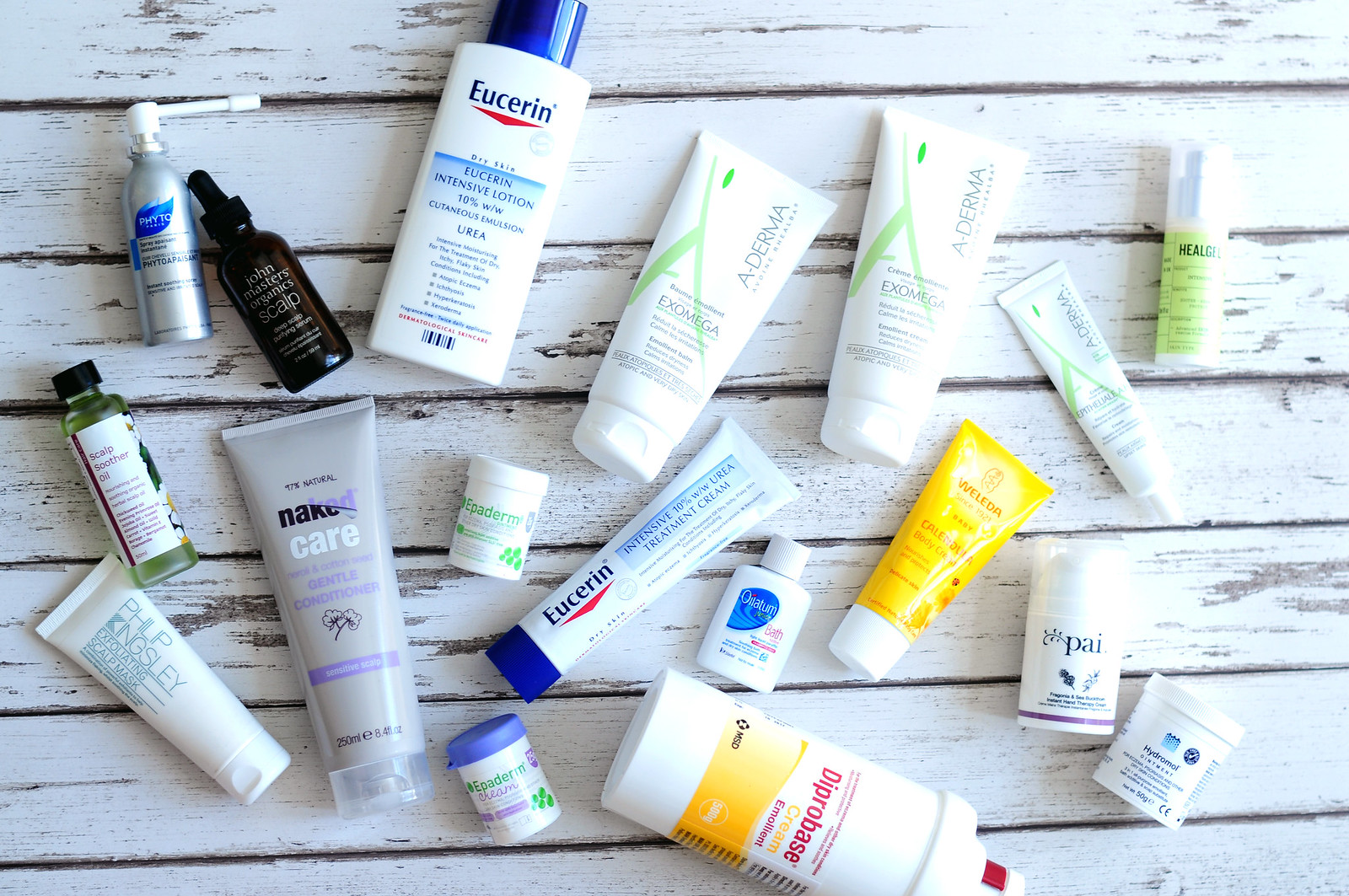In the image, a collection of skincare and wellness products is carefully arranged on a weathered, white wooden table, revealing hints of the wood's natural brown beneath the faded paint. The assortment includes various containers such as lotion bottles, creams, and ointments. Brands featured in this display include Eucerin, Naked Care, PAI, and A-Derma. On the upper left side, there is a small amber glass bottle with an eyedropper, labeled "John Masters" with some illegible text related to scalp care. Additionally, there is a glass bottle filled with green fluid, labeled as a scalp soother, positioned to the left. 

Towards the far right, a cylindrical tube with a green label stands out, highlighted by bright light on one side. In the middle of the arrangement, there is a striking bottle with a flat top and a bright yellow, round lid. This bottle is flanked by two slightly larger white bottles with similar shapes, featuring green patterns nearby. The detailed and eclectic mix of products suggests a well-rounded approach to personal care and wellness.